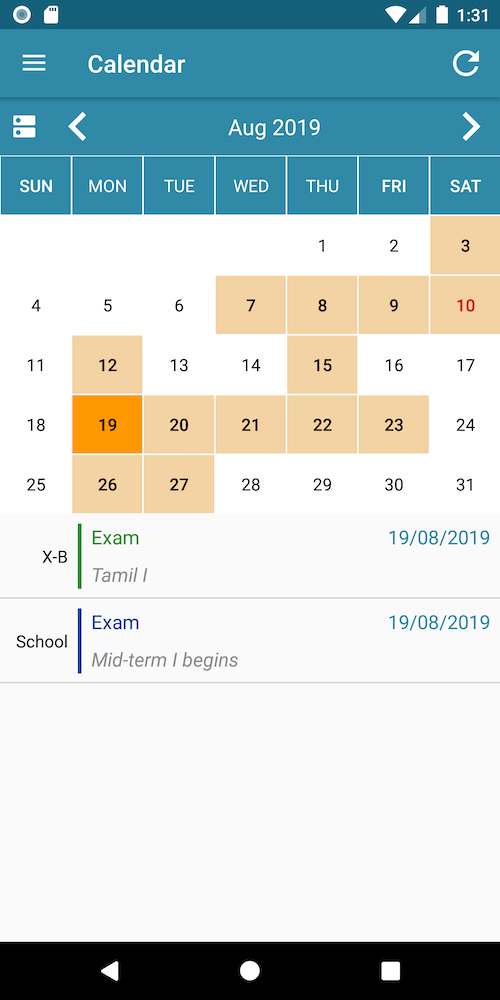This screenshot showcases a mobile application, likely running on Android given the icon designs. At the top left, there's a circular record button with a white border and navy blue center. To its right, a white SIM card icon is present. Adjacent to that, on the far right, are the Wi-Fi signal and cellular reception icons, both in white, with the cellular bar half-filled. The battery icon, fully white and filled, indicates a full charge, while the time displayed is 1:31.

Below this top bar, the interface features a calendar with a light blue background and white text. On the top left of the calendar is a settings icon represented by three stacked white lines. On the opposite end, an icon for refreshing the page is visible. The calendar displays "August 2019" prominently in the center, flanked by back and forward arrow buttons to navigate between months. The days of the week, from Sunday to Saturday, are listed, with Thursday marking "August 1" and continuing through to "August 31," which falls on a Saturday.

Within the calendar grid, notable dates are highlighted in green text. For instance, "Exam for Tamil I" is noted, with "X-B" preceding it on the left. Each event is paired with a date stamp on the extreme right, formatted as "19/08/2019." Another event titled "Midterm I begins" is listed below, accompanied by "school" on the left and the same date stamp format on the right (19/08/2019).